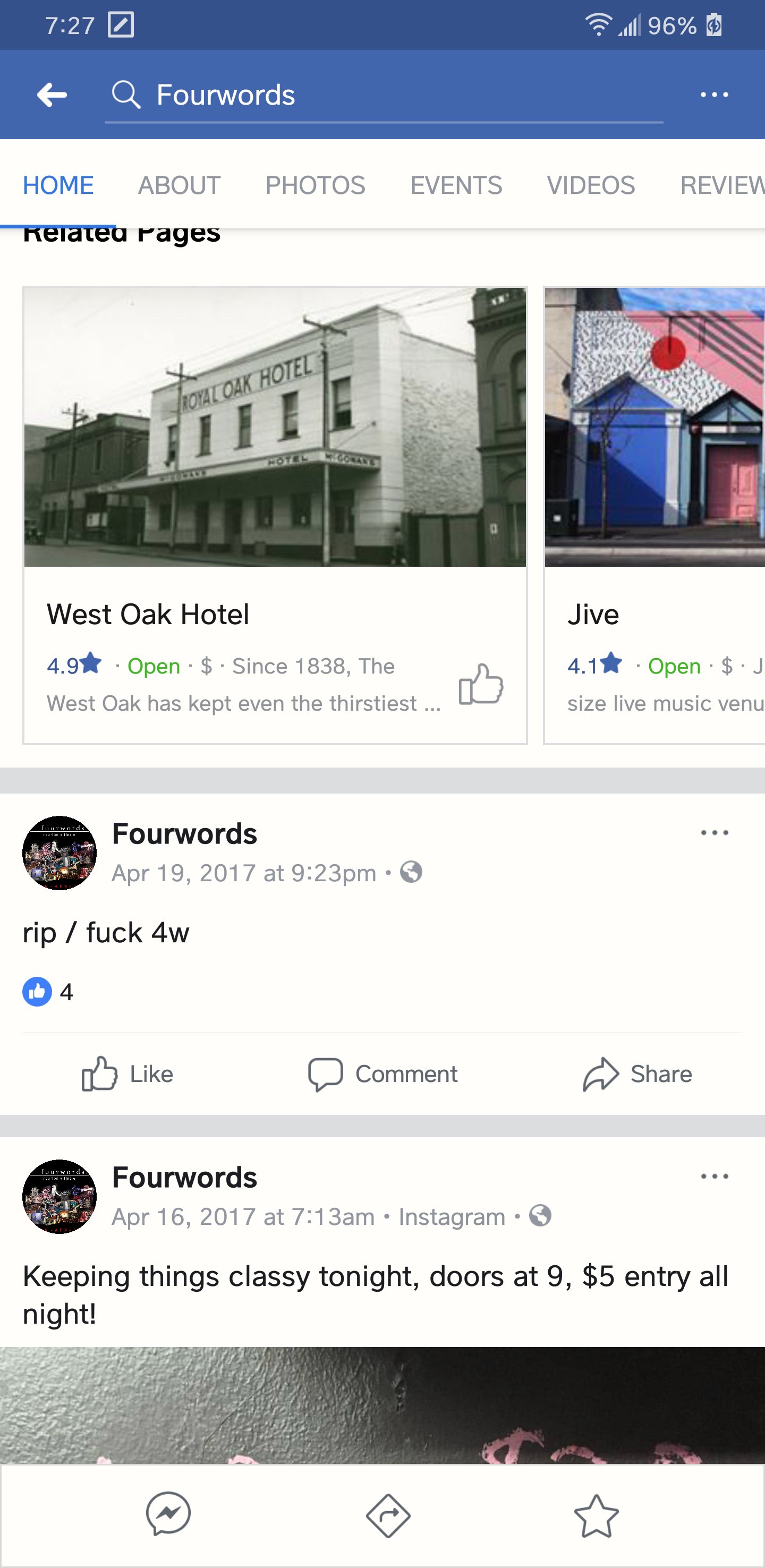This is a detailed screenshot of a mobile phone displaying a social media feed that resembles a Facebook layout. At the top of the phone screen, the time is shown as 7:27 along with the Wi-Fi signal, 4G mobile signal, a battery level of 96% with a charging icon. The app screen has a header with a search bar, a back button on the left, and three dots indicating a settings menu on the right.

The current page is dedicated to an account named "4Words," presented in a light blue color scheme typical of Facebook. Primary navigation tabs are visible and labeled: Home, About, Photos, Events, Video, and Reviews. Below these tabs are small preview cards of related pages, Westhawk Hotel and Jive, showing their status and opening times, with a thumbs-up icon for liking the pages.

Further down, there are two posts from the "4Words" account. The first post reads, "RIP / fuck4w" and has received four likes. The second post, "Keeping things classy tonight, doors at 9, $5 entry all night," appears just below, with a partially visible image that is too cropped to identify but suggests a nightlife or club scene.